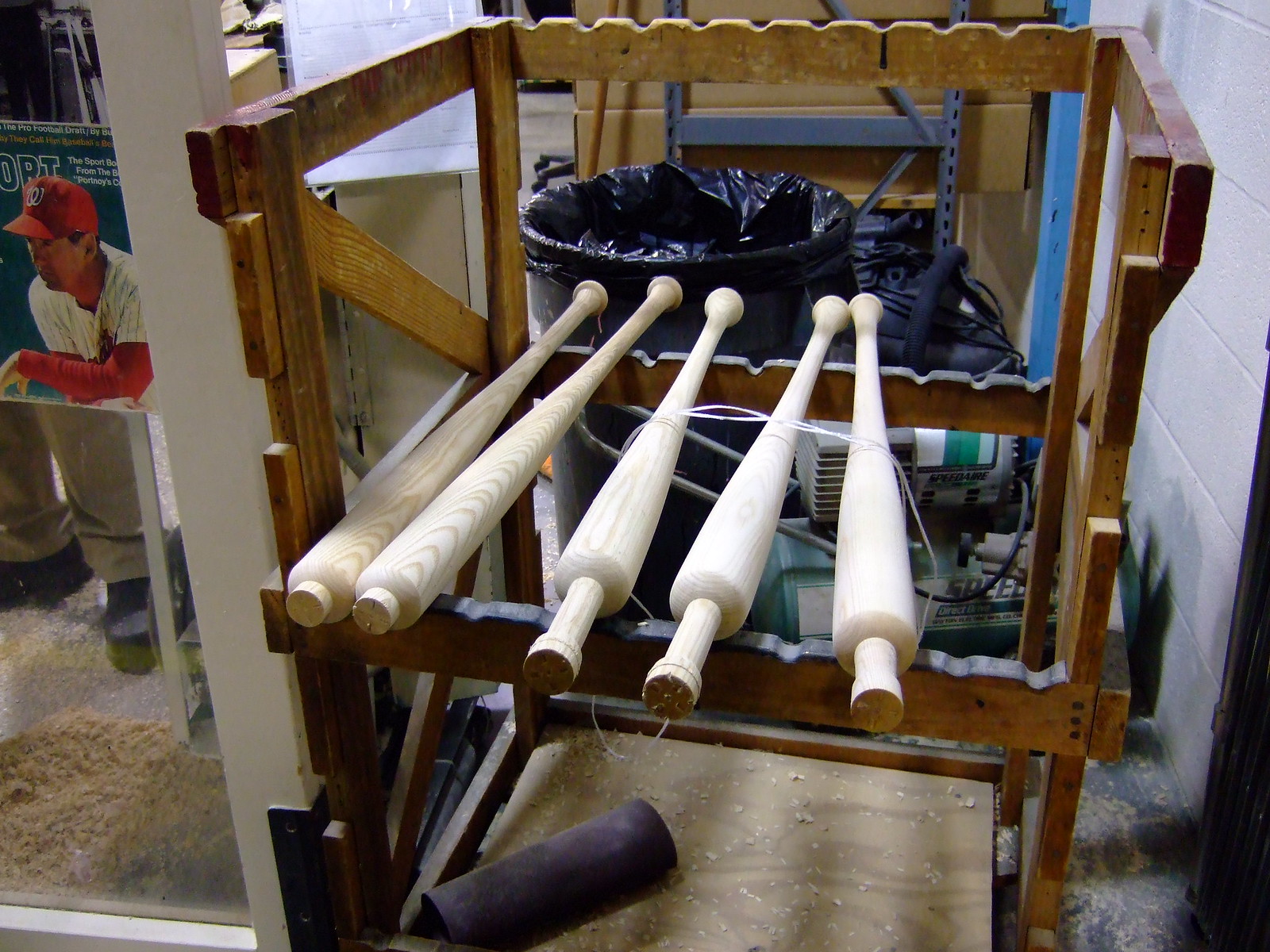The image depicts a bustling workshop dedicated to the creation of baseball bats. At the center, five wooden bats are in varying stages of completion, all resting on a dark wooden stand comprised of slatted supports. These unfinished bats, with their characteristic handles and widening barrels, still have small nubs of wood protruding from their ends, indicating they need further refinement. Below the bats, a purple roll of material, potentially sandpaper or rubber, is visible. The floor beneath them, likely concrete, is scattered with a pile of wood shavings and marked by a faint yellow safety line. Off to the left, a photo of a baseball player dressed in a pinstriped uniform and sporting a Wilson hat adds a touch of authenticity and inspiration to the space. Nearby, the black shoes of a worker can be seen, along with a trash can lined with a black trash bag. The detailed scene captures the meticulous craftsmanship involved in bat-making amidst a clearly organized and safety-conscious workshop.